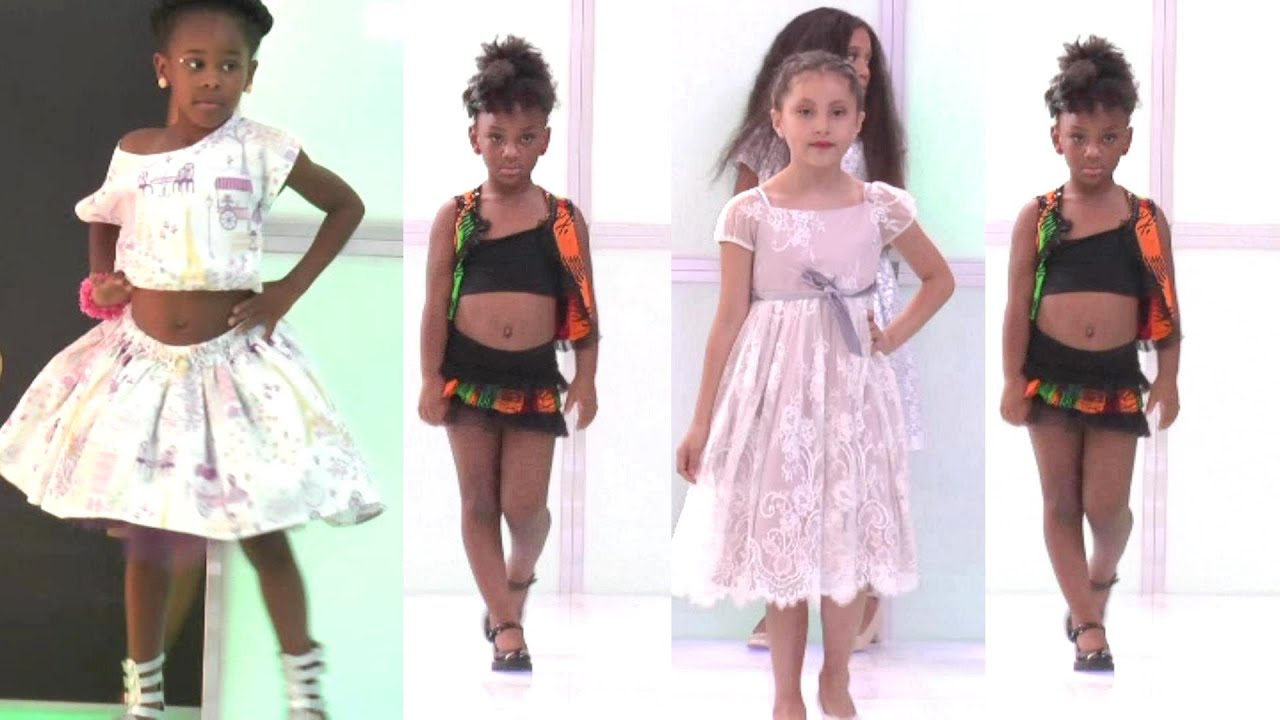This series of color photographs showcases a group of young girl models, likely around the ages of 9 or 10, participating in what looks like a fashion show, potentially on a runway. The first image features an African-American girl wearing a white two-piece outfit: a puffy, knee-length skirt adorned with a printed pattern of pink carriages and a matching off-the-shoulder crop top. She accessorizes her look with strappy white sandals, earrings, and a pink scrunchie on her right arm. 

The second girl, also African-American, is dressed in a striking black and orange two-piece ensemble. Her outfit includes a crop top, a black skirt with colorful tulle, and a coordinating jacket. She is seen in dressy black shoes.

The third girl, with medium-toned skin, wears a conservative knee-length light pink dress with short sleeves and lace detailing. Her hair is pulled up, and she is sporting red lipstick. There is another female figure, possibly her mother, standing behind her.

The fourth image is a repeat of the second girl in the black and orange outfit, confirming the emphasis on her striking ensemble. Altogether, these four images highlight the distinct styles and presentation of the young models, with a repetition that draws additional attention to specific designs.